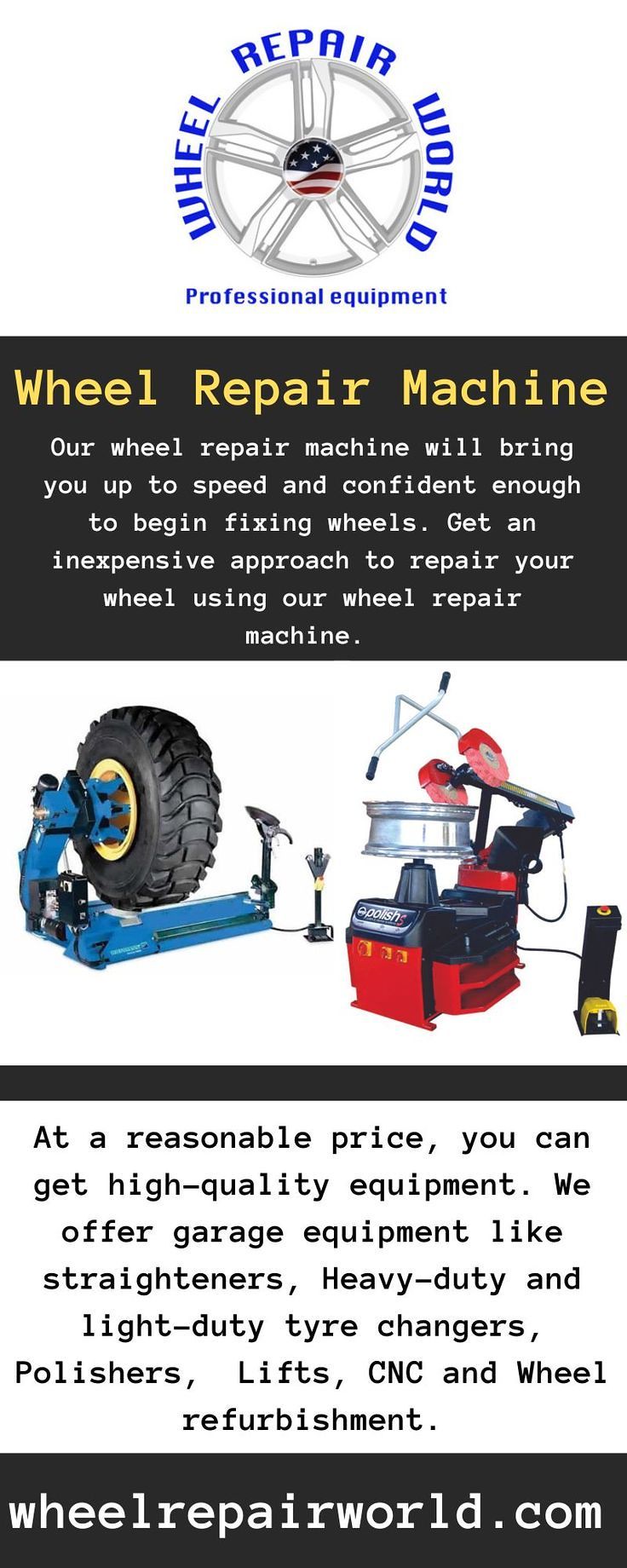The image is an advertisement for Wheel Repair World. The flyer is rectangular, aligned horizontally. At the top, set against a white background, is a silver hub cap with an American flag in the middle. Surrounding it, in blue text, are the words "Wheel Repair World Professional Equipment."

Beneath this, there's a gray box featuring yellow text that reads "Wheel Repair Machine," followed by white text that says, "Our Wheel Repair Machine will bring you up to speed and make you confident enough to begin fixing wheels. Get an inexpensive approach to repair your wheels using our Wheel Repair Machine." Below this description, the flyer presents images of two repair machines: a blue machine holding a fully rubber tire and a red one with a silver rim.

Next, on a white background with black text, it states, "At a reasonable price, you can get high-quality equipment. We offer garage equipment like straighteners, heavy-duty and light-duty tire (spelled as "T-Y-R-E") changers, polishers, lifts, CNC, and wheel refurbishment."

At the bottom, a thin gray bar contains white text that says, "WheelRepairWorld.com."